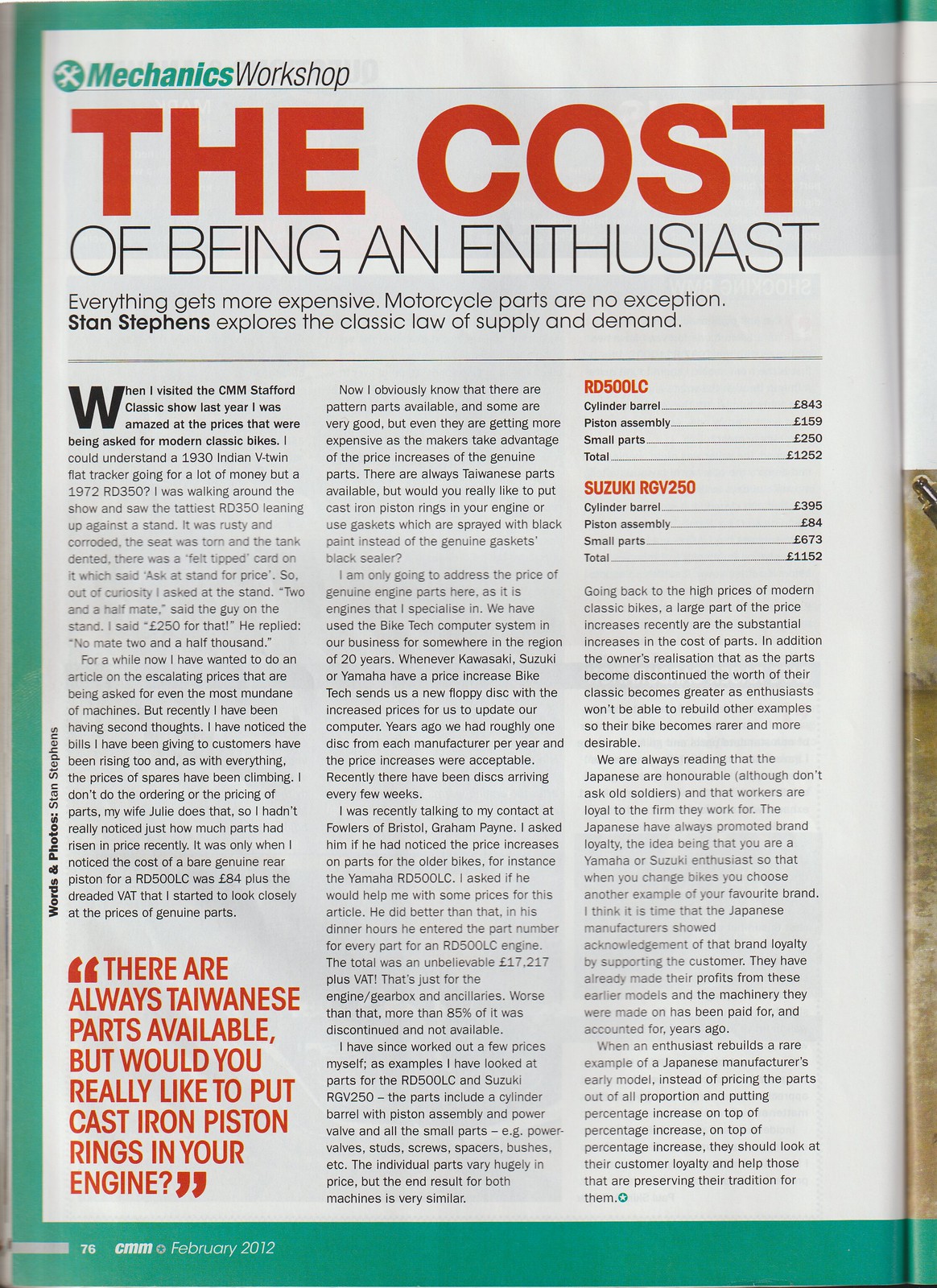This is a scanned page from a February 2012 issue of CMM magazine, specifically from the "Mechanics Workshop" section. The page features a green border on the top, left, and bottom sides. The title of the article, "The Cost of Being an Enthusiast," is prominently displayed at the top center with the words "The Cost" in bold red letters and "of Being an Enthusiast" in black. To the left of the title, "Mechanics Workshop" is written with "Mechanics" in green and "Workshop" in black.

Beneath the title, the subheading reads: "Everything gets more expensive. Motorcycle parts are no exception. Stan Stephens explores the classic law of supply and demand." The main body of the article is divided into three columns of text in a standard magazine font, mostly in black with occasional red highlights for emphasis.

The article discusses the rising costs of motorcycle parts, illustrated with personal anecdotes and specific examples. One notable story details the author’s shock at the high prices of modern classic bikes at the CMM Stanford Classic Show. There is also a highlighted inset quote in red capital letters at the bottom of the first column: "THERE ARE ALWAYS TAIWANESE PARTS AVAILABLE BUT WOULD YOU REALLY LIKE TO PUT CAST IRON PISTON RINGS IN YOUR ENGINE?"

At the top of the third column, a chart is presented with red headings that break down the costs of specific parts for two motorcycles—an RD500LC and a Suzuki RGV250. The chart lists prices like £843 for an RD500LC cylinder barrel and £395 for a Suzuki RGV250 cylinder barrel, highlighting the substantial expenses involved.

The text delves into the impact of these price increases on enthusiasts and the classic motorcycle market, criticizing manufacturers for not adequately supporting their loyal customers. The narrative emphasizes the escalating costs of genuine parts and the complexities of maintaining classic motorcycles in the face of these economic pressures.

The page is framed by a teal border around the edge, enhancing its visual appeal and distinguishing it within the magazine.